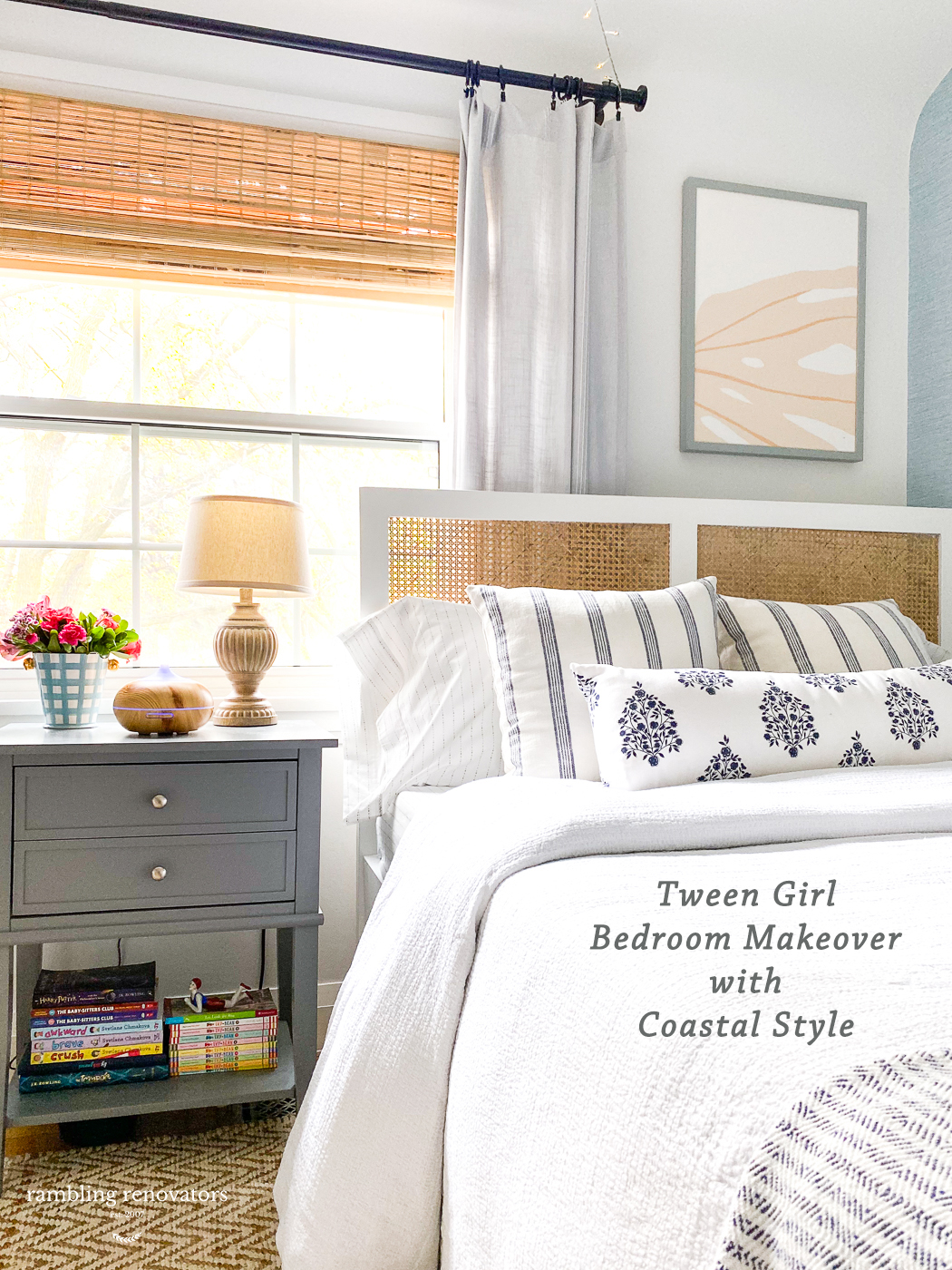This advertisement image showcases a computer-generated bedroom, specifically designed for a tween girl, with a coastal style theme. In the bottom right corner, the text reads "Tween Girl Bedroom Makeover with Coastal Style."

The focal point of the room is the bed, which is slightly offset to the right. The bed features a white comforter adorned with blue stripes and a variety of pillows, including a large rectangular body pillow with a black, tree-like dot design, and two large white and gray-striped pillows. The bed’s headboard has a white frame with tan wicker paneling. The wall behind the bed is painted in a light grayish-blue color.

To the left of the bed stands a gray nightstand with two drawers and a bottom shelf holding two piles of books. On top of the nightstand, there is a tan-colored table lamp, a small round object, and a vase with a bouquet of pink roses. 

A large window, framed in white, allows sunlight to flood into the room. It has a black curtain rod with white curtains pulled back, revealing rolled-up bamboo blinds. 

Finally, above the bed on the right side, a plain-framed painting with white and orange hues adds a touch of minimalistic decor.